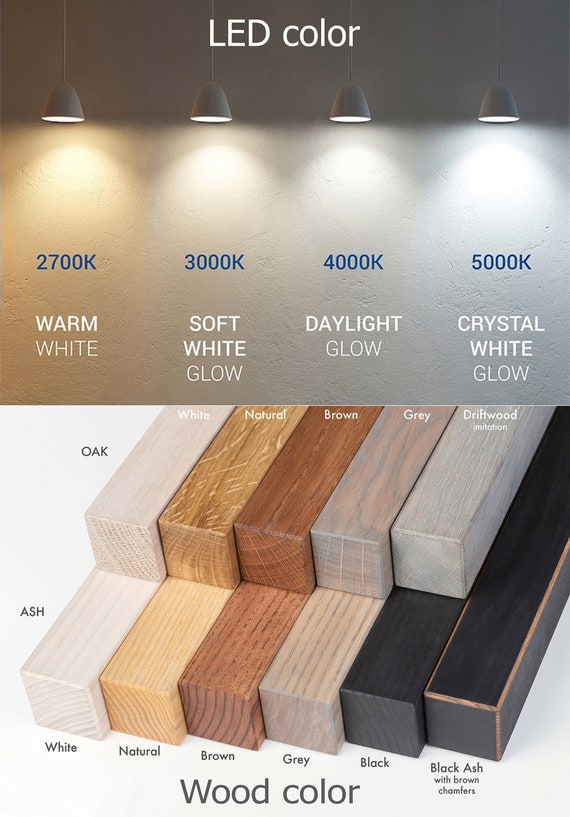The image is a full-color advertisement comprised of two distinct sections. The upper section features a display of four white pendant lamps hanging from the ceiling against a white wall background, each illuminating with a different type of light bulb. The text "LED Color" is prominently displayed at the top in white. Each lamp is labeled with its corresponding LED color temperature and description: 2,700K (warm white), 3,000K (soft white glow), 4,000K (daylight glow), and 5,000K (crystal white glow). The lower section showcases a selection of rectangular wood pieces stacked in two rows. These pieces gradate from lightest to darkest, representing different wood stains. The wood colors are labeled as oak, white, natural, brown, gray, driftwood, black, and black ash. Additionally, the text "Wood Color" is written in black at the bottom of this section, highlighting the variety in wood stain options. The two sections together provide a comprehensive view of LED light shades and wood color stains for potential buyers.